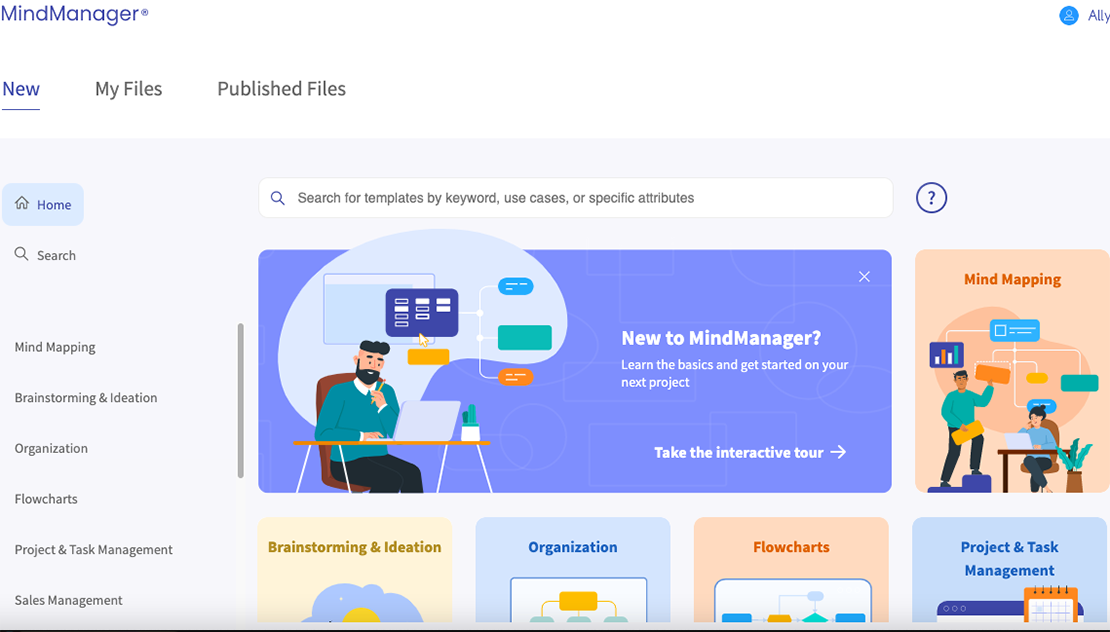Screenshot of the "Mind Manager" Website:

The screenshot captures a detailed view of the "Mind Manager" website. 

**Top Navigation:**
- **Top Left:** The website name "Mind Manager" is prominently displayed in a purple font. Directly beneath this, the title of the current page is oriented.
- **Top Right:** A small circle contains an outline of a blank profile picture next to the name "Ally" (spelled A-L-L-Y).

**Header Section:**
- Below the "Mind Manager" title, there are three header options with drop-down menus: "New" (underlined to indicate it's active), "My Files," and "Publish Files."

**Sidebar Navigation (Left Column):**
- A scrollable list of navigation items is arranged vertically:
  - **Home** (icon: house)
  - **Search** (icon: magnifying glass)
  - Between sections, there is a small amount of space for clarity.
  - Various sections listed are:
    - Mind Mapping
    - Brainstorming and Ideation
    - Organization
    - Flowcharts
    - Project and Task Management
    - Sales Management

**Main Content Area (Right):**
- The main section is populated with colorful, cartoonish tiles:
  - A large purple rectangular tile featuring a cartoon man sitting at a desk. The text reads: "New to Mind Manager? Learn the basics and get started on your next project. Take the interactive tour," accompanied by a clickable button with an arrow.
  - Smaller tiles surround the main tile, each depicting distinct sections listed in the sidebar with corresponding cartoonish and colorful designs.

The layout organizes information in a user-friendly manner, with a clear hierarchy for easy navigation and access to various tools and features.